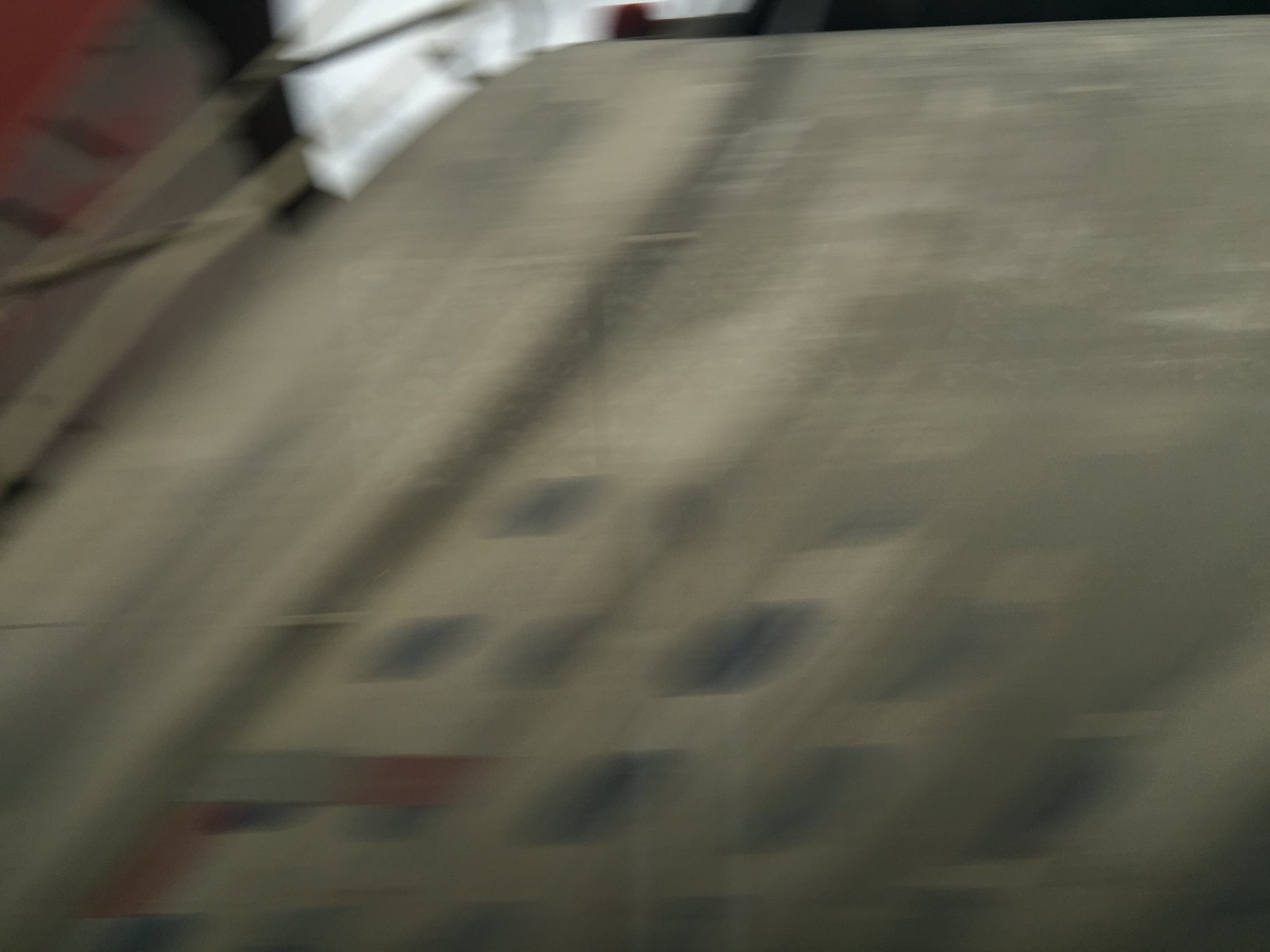This image is a very blurry photo that is difficult to discern. It appears to capture a flat surface, possibly the floor, with some debate over whether it might also be carpet with an ornate design featuring blue squares and gray streaks. A white area in the image could be part of the floor, wall, or even a piece of furniture like a fallen chair in the upper left corner. Additionally, there is some red coloring seen in the upper left portion, potentially suggesting a trick of the light, an object, or just a distortion. Overall, it seems like an accidental photo likely taken by someone who was moving, making it hard to clearly identify the subject.